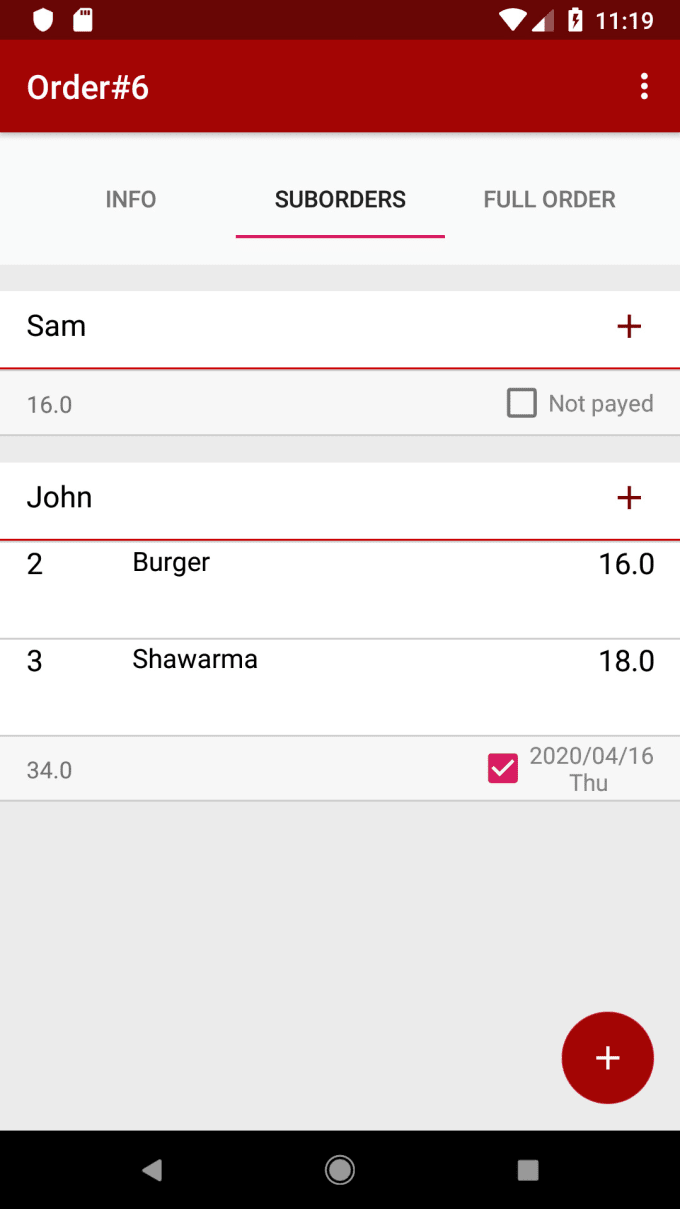This screenshot from a food delivery app features a detailed interface for managing an order. At the top of the screenshot, a maroon bar displays "Order Number 6" in white font at the top left corner. To the far right of the bar, there is a three-dot icon indicating additional options. 

Below the maroon bar, there are three categories listed horizontally: "Info," "Sub Orders," and "Full Order." Beneath these tabs, the name "Sam" is displayed on the left side, immediately followed by a plus sign "+" on the right. 

The text "16.0" appears underneath "Sam," adjacent to an unchecked square checkbox labeled "Not Paid." Below this section, the details of the order are provided: 
- "John: Two Burgers 16.0"
- "Three Shawarma 8"

Further down, the total amount "34.0" is noted in small black numbers to the right, accompanied by a checked checkbox. The date section follows, indicating "Thursday" (abbreviated as "Thu"). 

In the bottom right corner of the screenshot, there is a red circle with a white plus sign in the center, likely a button for adding items or actions related to the order.